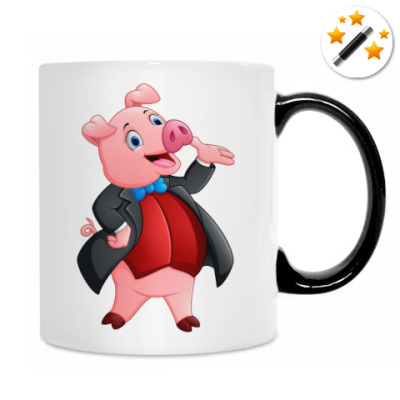The image depicts a white coffee mug with a black, rounded handle positioned on the right side. Against a white background, the mug features a detailed illustration of a pink pig dressed in a sophisticated outfit. The pig wears a black suit jacket, a sky blue bow tie, and a red vest. The pig's head is tilted up and to the side, smiling with big eyes. Its left hand is raised with the palm facing up, while the right hand is placed on its hip, and a small curly pink tail peeks out from behind. Additionally, the pig's hooves are a darker red color. In the upper right corner of the image, there is a white circular button containing five gold stars of various sizes, two small, one medium, and two larger, alongside a mysterious cylindrical object with black and silver segments.